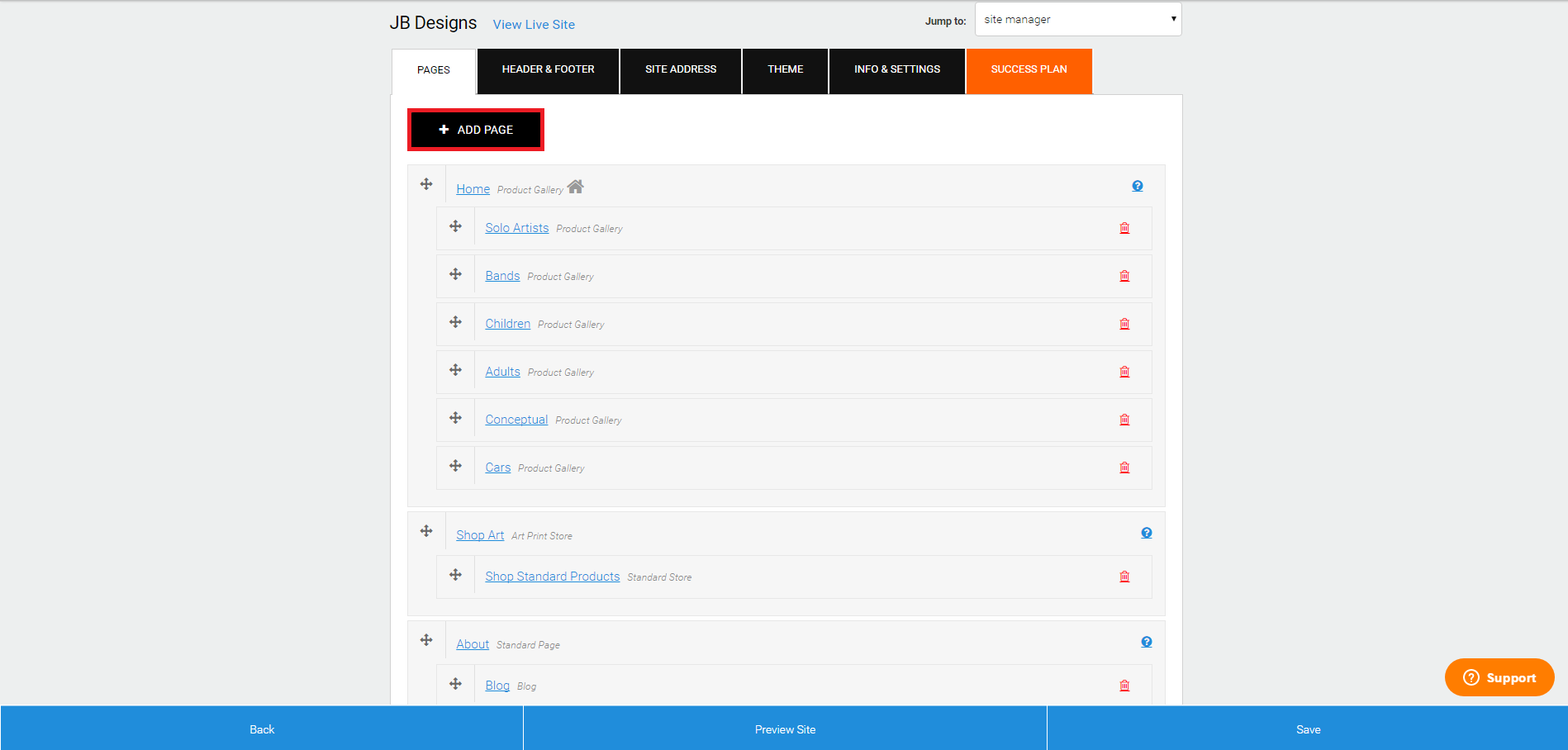The image depicts a web page from a web design platform named 'JB Designs'. At the top left corner of the page, 'JB Designs' is prominently displayed in bold black lettering. Adjacent to this, in smaller blue letters, the text 'View Live Site' is visible.

On the top right of the page, there is an option labeled 'Jump To' with a drop-down menu set to 'Site Manager'. The exact options available in the drop-down menu are unspecified.

Below this top navigation bar, various tabs are organized horizontally across the page, each with a brown background and white lettering. The tabs include 'Header and Footer', 'Site Address', 'Theme', 'Info and Settings', and a bright orange tab labeled 'Success Plan'.

Directly beneath these tabs, a row features an orange rectangular box with a white plus sign, accompanied by the text 'Add Page'. Below this button, a list of additional pages that can be added is displayed: Home Page, Solo Artists, Bands, Children, Adults, Conceptual, Cars, Shop Art, Shop Standard Products, About, and Blog.

At the bottom of the page, a blue bar with three sections offers further control options labeled 'Back', 'Preview Site', and 'Save'. An orange button for 'Support' is also present, indicating assistance is available for users creating their web pages.

Overall, this image appears to be a screenshot from a web design platform, offering various tools and options for building and managing a website.